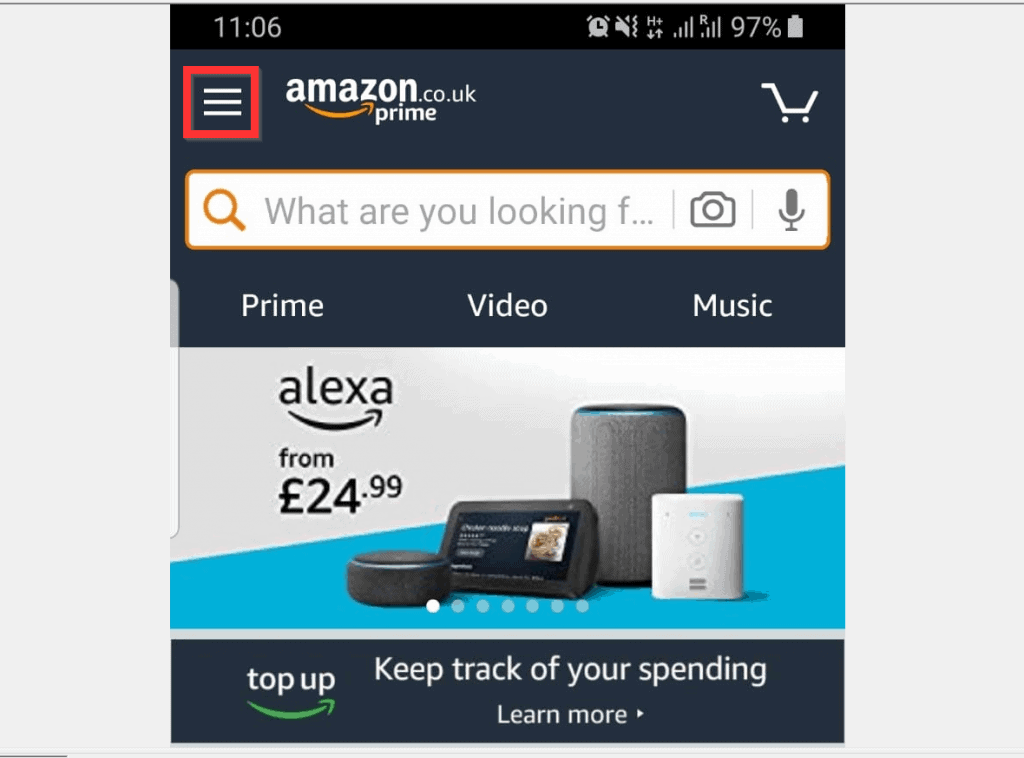This image is a detailed screenshot taken from a cell phone displaying the Amazon UK mobile app interface. The screenshot was captured at 11:06 AM, as indicated by the clock on the top bar, which also shows icons for an alarm clock, vibration mode, and a battery level at 97%. 

At the very top left, there are three horizontal lines, encapsulated within a red square. To the right of this, it reads "Amazon.co.uk" followed by a Prime logo. On the top right of the screen is a white shopping cart icon. 

Below this, the interface features a prominent rectangular search bar, which has an orange magnifying glass icon on the left side and the placeholder text "What are you looking for?" Inside the search bar, there's also a camera icon and a microphone icon to the right. 

The next section below the search bar highlights some promotional content, starting with the labels "Prime Video" and "Music". The main advertisement displayed is for Alexa-enabled devices, depicted in a photograph. The promotion indicates that these devices are available starting at £24.99. 

Additionally, there are prompts for users to "Top up, keep track of your spending, learn more," all situated within the same promotional section.

The screenshot is displayed against a plain white background. There are no people, animals, plants, flowers, trees, buildings, or automobiles present in the image.